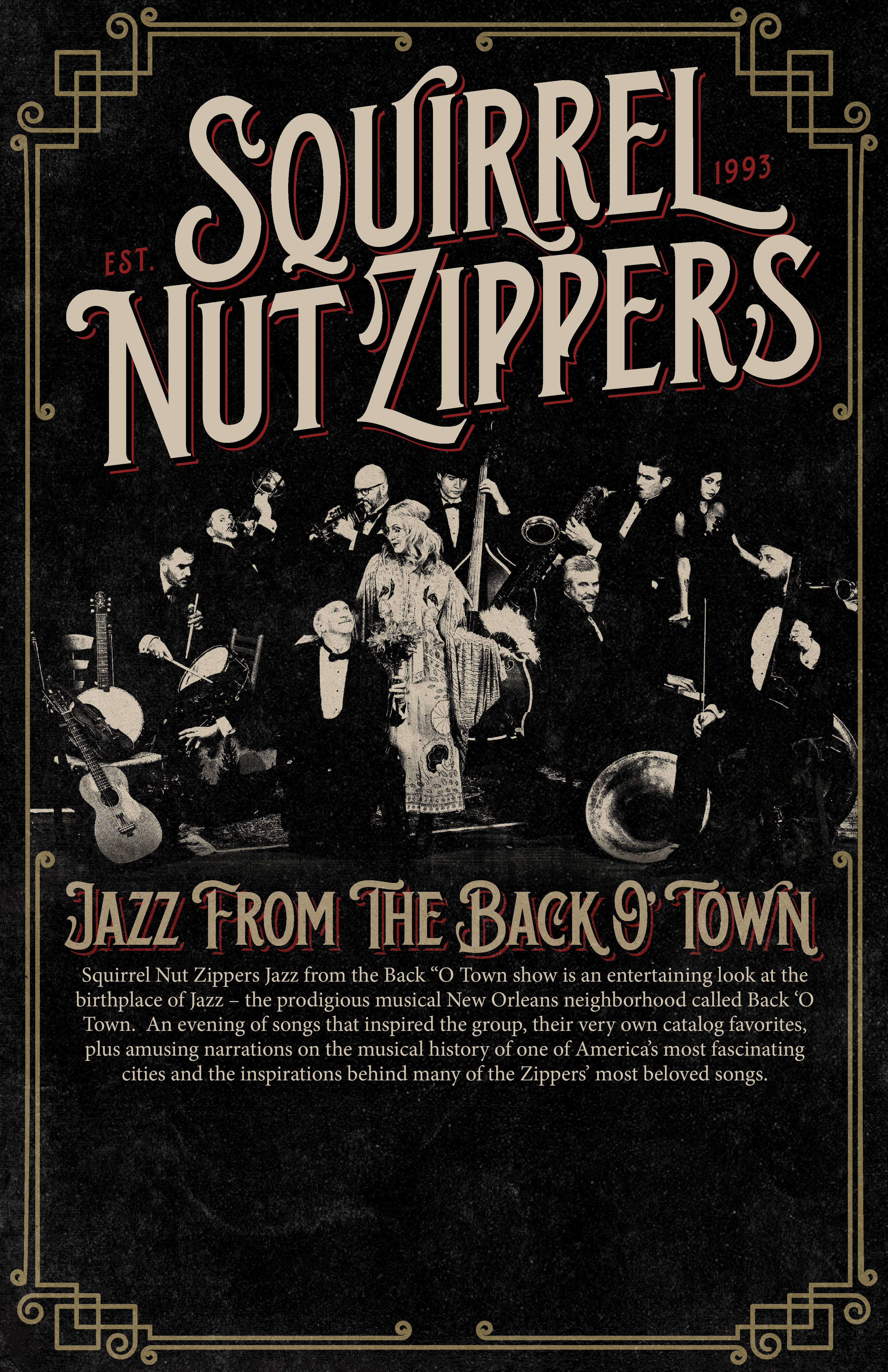This image is a stylized, vertical concert poster advertising the jazz band Squirrel Nut Zippers. The design features an ornate Art Deco border with elegant, filigree detail, predominantly in black with text in pale beige and yellow. At the top, in a striking, stylized typeface, it reads "Squirrel Nut Zippers, Established 1993." Below this header, the band members are depicted in a vintage black and white photograph evocative of the Big Band era.

The ensemble consists of approximately ten musicians, mostly gentlemen dressed in black tuxedos with white shirts and black ties. Central in the image is a woman in a 1920s flapper-style dress and headband, standing gracefully while looking at a gentleman who is kneeling and gazing up at her adoringly. The surrounding band members hold various musical instruments, including a guitar, bass, trombone, violin, and saxophone, reinforcing the lively jazz theme.

Beneath the photograph, in a smaller font, the text reads, "Jazz from the Back-O-Town," an homage to the prodigious New Orleans neighborhood renowned as a birthplace of jazz. Additional copy describes the "Squirrel Nut Zippers Jazz from the Back O-Town show" as an "entertaining look at the birthplace of jazz," highlighting it as an evening of songs that inspired the group alongside their catalog favorites, enriched by amusing narrations on the musical history of New Orleans and the inspirations behind many of the band’s beloved songs.